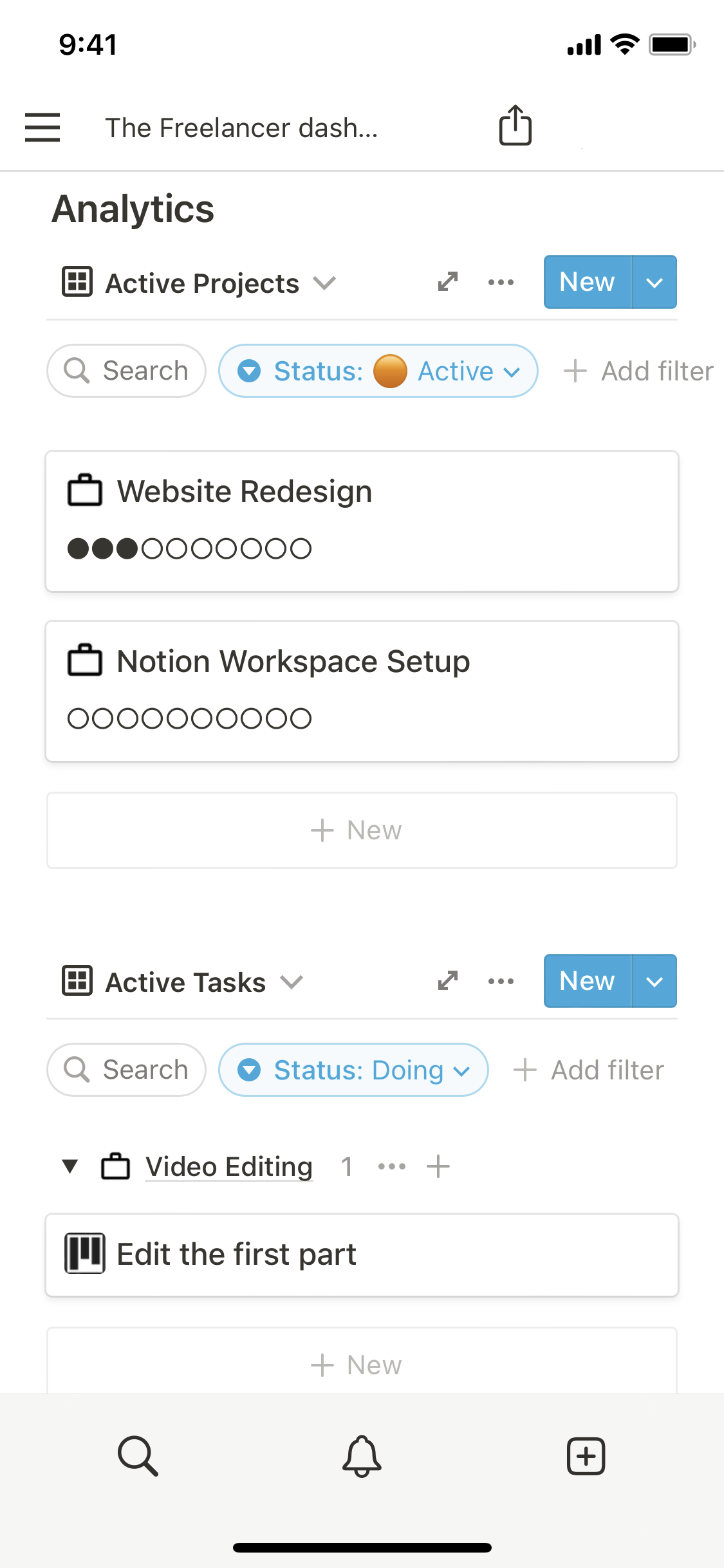Screenshot of a Freelancer App Dashboard Detailing Project Progress and Active Tasks:

The image displays a detailed view of a Freelancer app dashboard that offers comprehensive analytics reports for both active and inactive projects. At the top of the screen, the "Website Redesign" project is highlighted under the active reports section, showing that it is less than halfway completed. Another project, "Notion Workspace Setup," is also listed but remains entirely unstarted. 

Moving on to the active tasks section, the dashboard indicates an incomplete task related to video editing, which the user has not progressed on. Below this, another task is listed, but the exact details are truncated; however, the app prominently prompts the user to edit this initial section.

The interface at the bottom of the screen features a search bar icon for quick navigation, a bell icon to signify notifications or alarms, and an additional icon that allows users to add new projects or tasks, or apply filters to manage their workload more effectively.